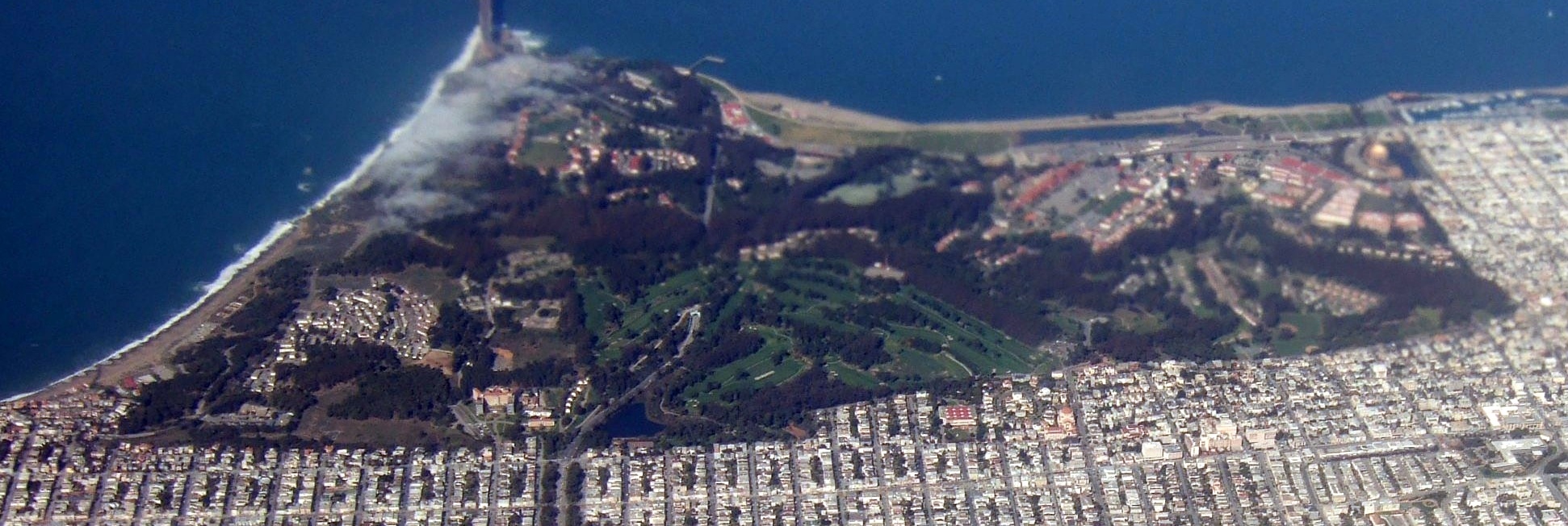The image depicts an aerial view of a coastal region, likely a peninsula, showcasing a mix of urban development and natural landscape. The scene includes numerous small houses scattered throughout, with some sections visibly dark and brown, possibly resulting from a destructive event, such as the Hawaii fires. Surrounding these areas are untouched houses, lush green patches of grass and trees, and the blue ocean with waves crashing onto the beach. There are some red dots, presumably rooftops, adding to the vibrancy of the view. The housing stretches from the bottom left corner of the image moving right and upwards, contrasting against areas of significant greenery and forest. The image lacks any textual elements and is marked by a palette of dark browns, blacks, greens, blues, whites, and hints of red. It appears to be formatted in a way that might suit a website header, capturing the juxtaposition of developed and natural spaces in a unique and visually compelling manner.